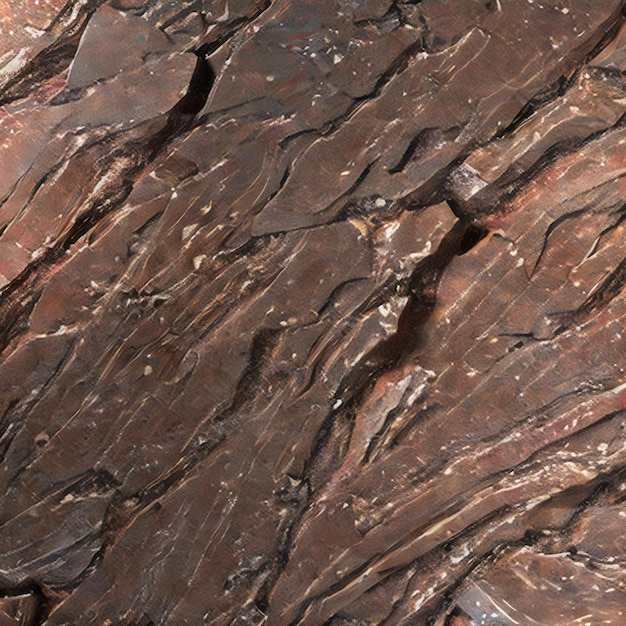This is a highly detailed close-up image of a weathered rock surface, perhaps magnified to emphasize its intricate details. The rock exhibits a rich palette of reddish-brown hues, reminiscent of copper, with varying shades from pale to saturated tones. The surface is primarily flat but interspersed with jagged crevices and striations, suggesting a natural formation that might have been shaped over time by elements such as water or wind. These irregular grooves and depressions give the rock texture, with the deepest and most prominent groove located in the top left corner, about four times deeper than the others. There's a noticeable gradient, with the browns becoming darker towards the center and lighter and more reddish at the edges. The rock's surface also features small white specks or pale light brown spots, possibly mineral deposits, adding to its weathered and aged appearance.